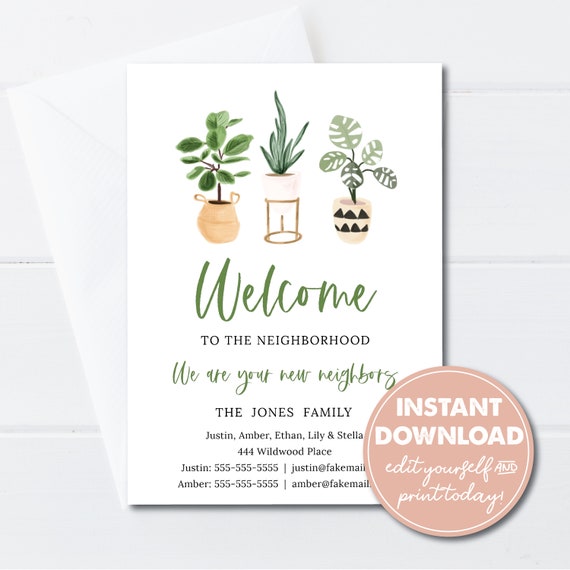This image features a high-quality digital mock-up of a "Welcome to the Neighborhood" card, designed to resemble an Etsy product. The card, adorned with a watercolor illustration of three potted plants—one in a tan vase with many petals, another in a white vase on a brown stand, and the third in a green pot with black triangles—sits atop a white envelope on a white tile background. The text on the card reads in green and black, "Welcome to the neighborhood. We are your new neighbors, the Jones family," followed by the names Justin, Amber, Ethan, Lily, and Stella, and their address, 444 Wildwood Place. Contact information includes Justin and Amber's identical phone numbers, 555-555-5555, and their respective email addresses, justin@fakemail.com and amber@fakemail.com. In the bottom right corner of the card, a peach-colored circle indicates "instant download," promoting the card as an editable and printable digital file.